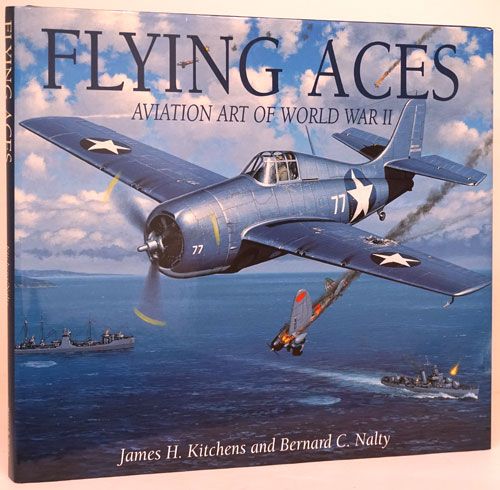The cover of the book features an artwork depicting an intense World War II air and sea battle scene. Dominating the center is a sleek, silver warplane with a propeller, flying to the left. The plane is adorned with dark blue circles on both its wings and fuselage, each containing a white star, and is marked with the number "77" in white print near the nose and on the side. Above the wings and beside the plane is the book's title in dark blue letters: "Flying Aces: Aviation Art of World War II." Beneath this title lies the subtitle and the authors' names: James H. Kitchens and Bernard C. Nolte.

The backdrop of the image showcases an oceanic battle. Below and behind the primary plane, a second aircraft, engulfed in flames and trailing dark smoke, spirals down towards the ocean. Scattered in the vast, blue sea are two large, gray battleships. The one in the bottom right corner is actively engaged in combat, firing its guns, with visible flames and muzzle flash. The sky above is a mix of blue and white, dotted with puffy clouds, adding a dramatic contrast to the chaotic battle below.